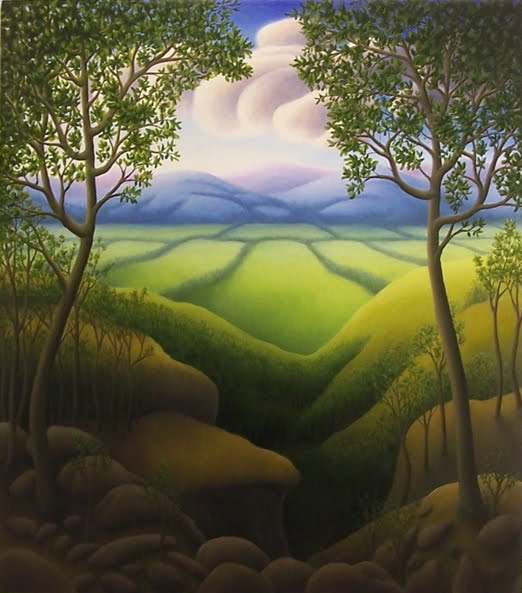The image depicts a computer-generated graphic of an outdoor scene showcasing green, rolling hills segmented by patches of land separated by darker green, taller plants, resembling hedges or wild grass. Framing the image are two main leafy trees that create an opening, revealing a slight gorge or dip in the landscape. Surrounding this dip are multiple smaller trees, descending into the darker central area. Beyond the foreground, the fields display a patchwork arrangement, defined by what appears to be low green hedges. In the background, a range of curved, round mountains or hills in hues of purple, blue, and pink form a scenic backdrop. The sky above features distinctive puffy clouds resembling marshmallows or glove hands. In the very foreground, rocks are scattered near a valley, adding texture to the scene. The overall color palette transitions from green in the midsection to darker yellow-brown tones towards the bottom.